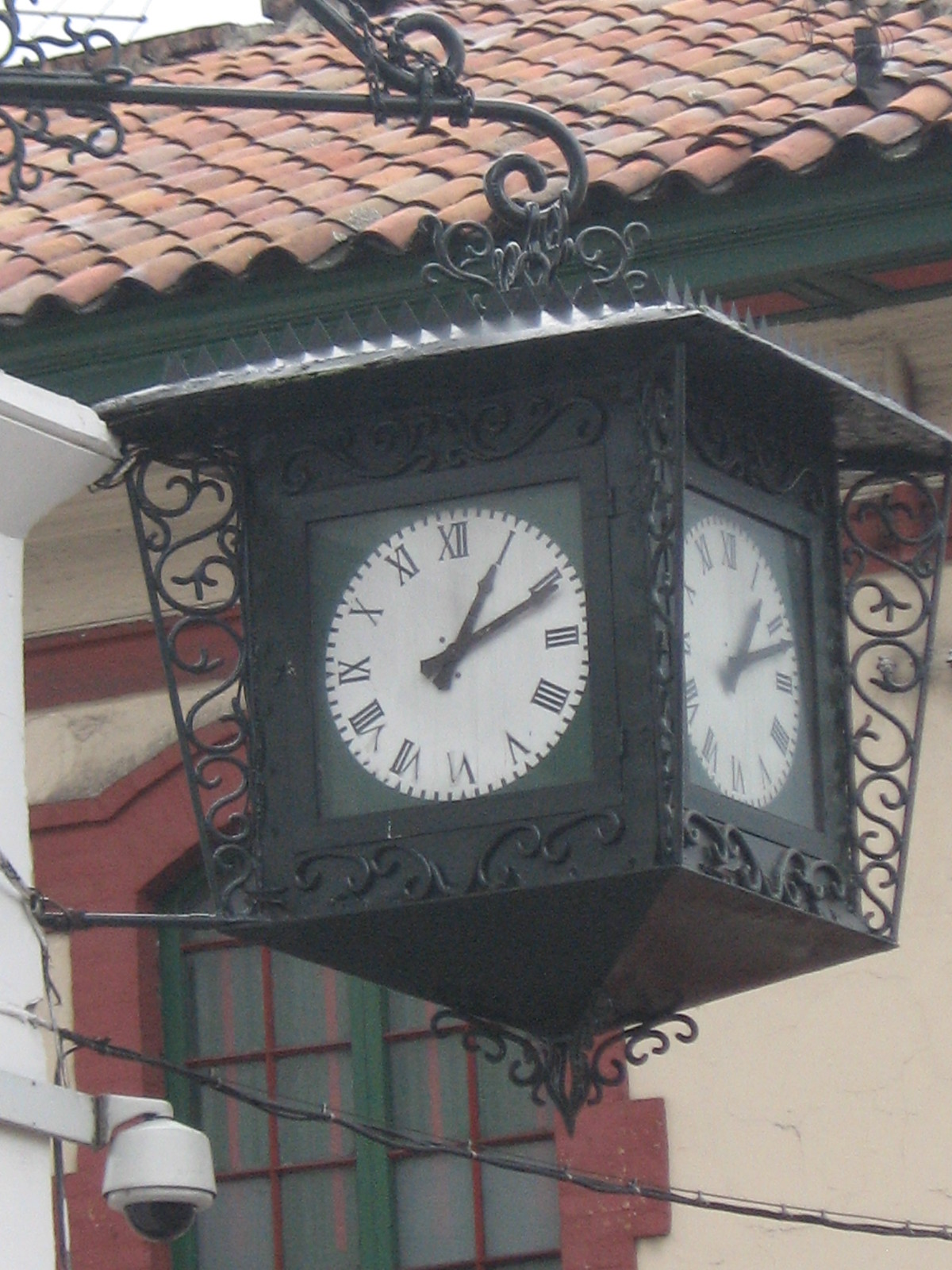The daytime photo captures the exterior of a beige stucco building with distinctive green-trimmed eaves and red brick outlining the large windows. Above the windows and near the roof, there's a prominent black cast-iron post adorned with ornate curlicues, supporting a large black square clock. Each side of this clock features a white face with black Roman numerals showing the time as 1:10, encircled by decorative metalwork. Below the clock, there is a street camera mounted on the same post. The roof is covered in reddish tiles, adding a touch of warmth to the scene. In the right corner, a rounded red light fixture protrudes from the wall, enhancing the building's intricate details. The photo showcases not just the clock's functional design but also the architectural nuances of the building.